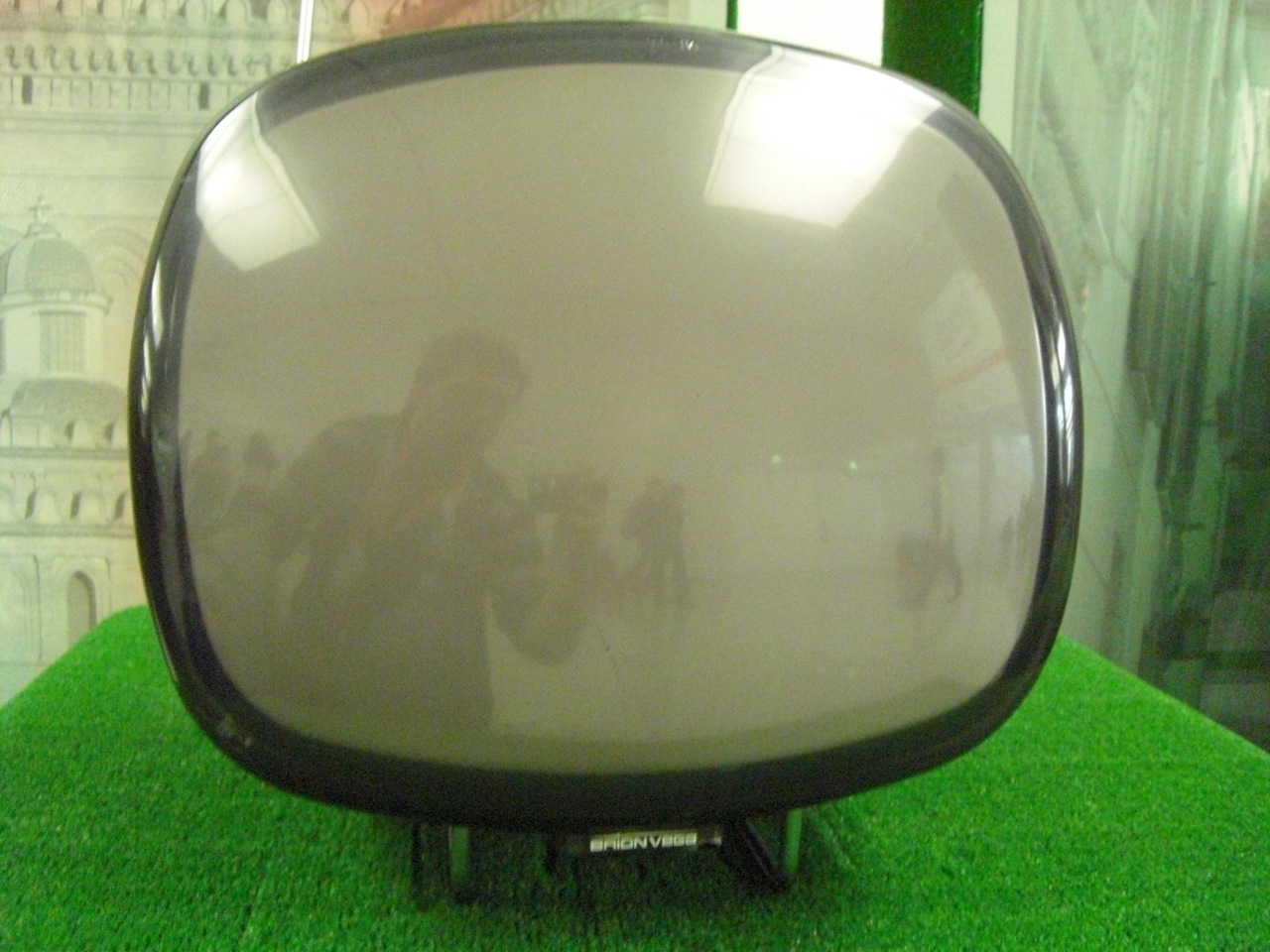The image showcases an object resembling an old television or possibly a vehicle headlight with a cloudy, whitish center, set in a black metal base. The object, more rounded than square, is positioned upright on a green felt or artificial turf stand. In its reflective surface, a young man is seen taking a photograph, along with vague reflections of fluorescent lights and other indistinct figures in the background. The base of the object is marked with a hard-to-decipher logo or text, potentially reading "Brian Vega" or "BRIONV2." The background features a white wall with a building's outline or shading on it. The image evokes curiosity about the object's identity and significance.